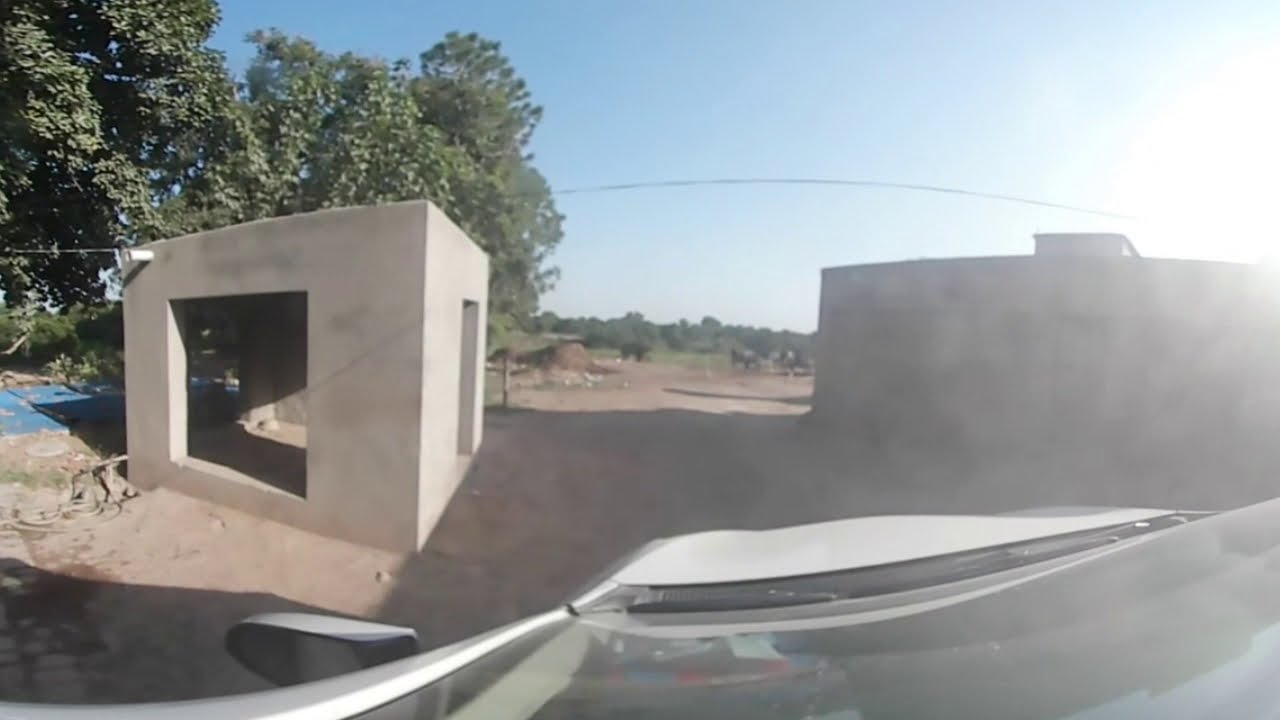This image, captured from the driver's seat of a white vehicle, presents a diverse scene through the left side of the windshield, as evidenced by the visible left rearview mirror in the lower left corner. The setting appears to be a daytime drive through a somewhat impoverished rural or semi-urban area, with bright blue skies and abundant sunlight casting glare across the scene.

In the foreground, just to the right of the vehicle's perspective, lies a square concrete or clay-like structure with large, open window cutouts. This box-like building is shaded under a canopy of tall trees standing prominently to the left. Adjacent to this, further right, stands another larger building, also giving the impression of being constructed from concrete or clay. Wires extend from the smaller structure towards the larger building, suggesting a functional connection between them. 

In front of these edifices, a dirt pathway stretches out, leading the eye towards the background where more dense trees populate the landscape. Along this dirt road, a tipped-over table or chair sits beside something blue on the ground, which could be a mat. In the far distance, beyond the trees and near the forested area, appear indistinct shapes of animals—potentially cows, horses, cattle, or perhaps even bears—seen grazing on the grass amidst the verdant expanse.

The detailed tableau painted by the interplay of architectural elements, natural scenery, and the presence of distant wildlife encapsulates a snapshot of a tranquil, albeit modest environment.